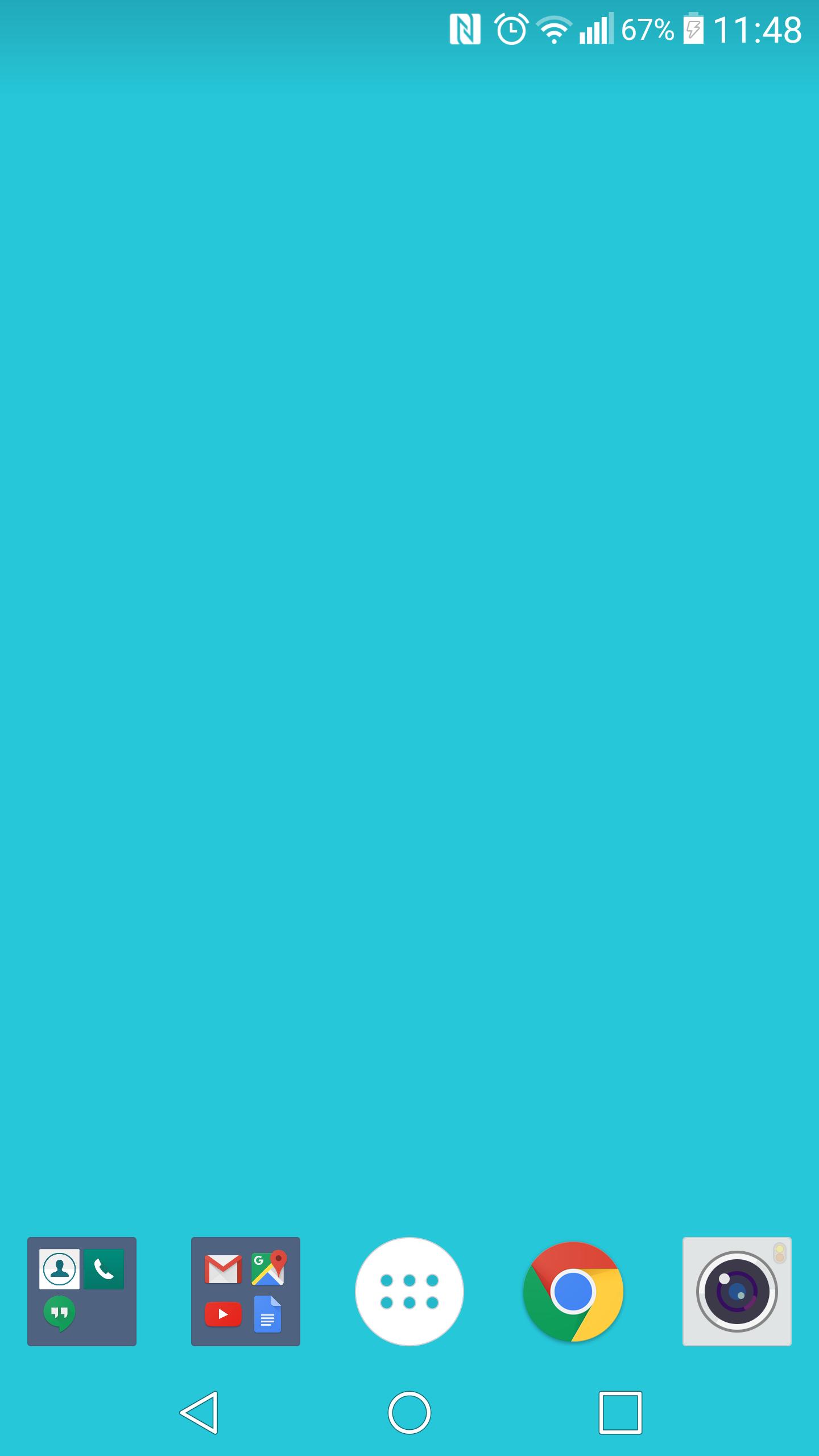This image features a screenshot taken from a tablet device. At the top-right corner, the time is displayed as 11:48, alongside a battery icon indicating 67% power remaining. The device also shows a telephony signal strength of four out of five bars and roughly three-quarters Wi-Fi connectivity. Additionally, a clock alarm icon is present, as well as an icon resembling a white rectangle with a blue letter "N" in it, whose specific function is unclear.

The main portion of the screen, approximately 80% of it, is a solid medium blue color devoid of any content. At the bottom of the screen, there are several folders and icons representing various apps and functionalities:

1. The first folder contains three icons: 
   - An icon likely for contacts.
   - An icon probably for telephone.
   - An icon that seems to represent a text messaging app.

2. The second folder houses four apps:
   - A Gmail app icon indicated by a red "M" on a white background.
   - A YouTube app icon characterized by a red play button.
   - A map app icon depicting a map.
   - An unidentified app icon represented by a blue folder with its top corner bent down on the right.

3. The third icon is a white oval with six dots, arranged in two rows of three, likely representing an app drawer or menu.

4. The fourth icon resembles a red, yellow, and green shutter with a blue dot in the middle, suggesting it might be for a camera or photo viewing app.

5. Next to it, there is a silver colored camera icon with a black lens and a blue spot in the center, hinting at a camera application.

At the very bottom of the screen, there are three navigational icons:
   - A left arrow triangle in white at the bottom-left corner.
   - A white oval in the center, indicative of a home button.
   - A white rectangle on the bottom-right corner, likely for accessing recent apps or multitasking.

Overall, this image captures the home screen of a tablet, providing an overview of available functionalities and connectivity status.